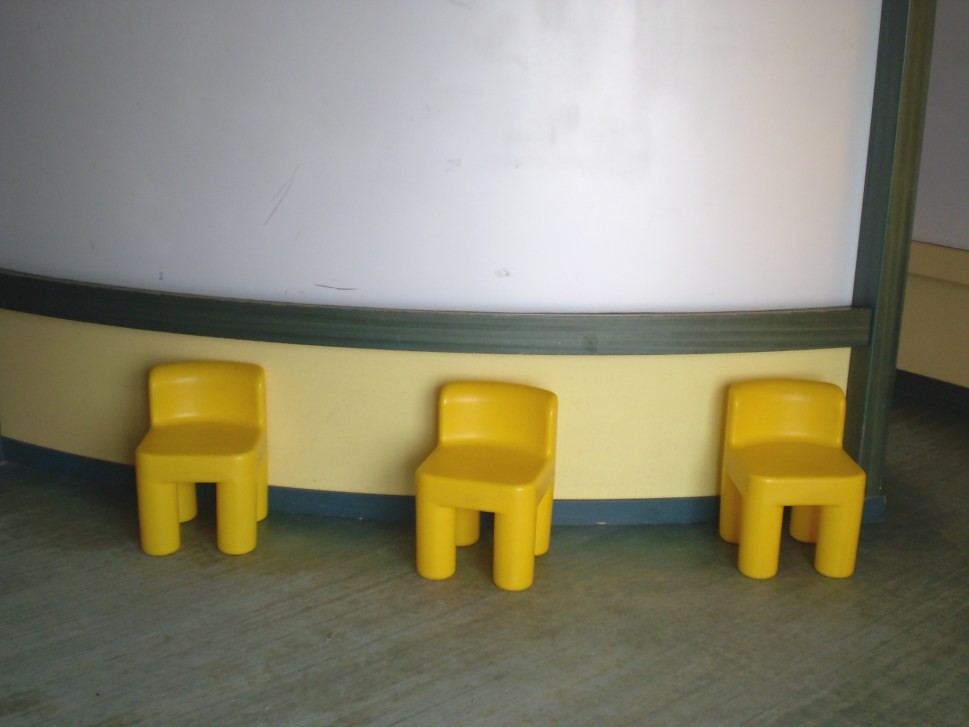This somewhat blurry color snapshot captures a section of a curved wall adorned with distinctive molding. The wall is segmented horizontally by thick wooden chair rails, possibly measuring around one by four inches, that follow its gentle curvature. Above the wood molding, the wall is painted white, while the area directly below it features a butter yellow hue. The baseboard further down is painted a dark blue or gray, providing a striking contrast.

Lined up against this wall are three small, vibrant, primary yellow children's chairs or stools, each with short legs resembling cylinders. The chairs are low to the ground, designed likely for toddlers, and are positioned in a slight arc. There are no pictures on the wall, lending a minimalistic feel to the composition.

The floor is a grayish, brownish-gray wood, adding to the understated color palette. Light streams in from the right, creating reflections on the white section of the wall and casting shadows, suggesting a nearby window. The photograph highlights a simple, bright, and well-structured room, designed thoughtfully for young children.